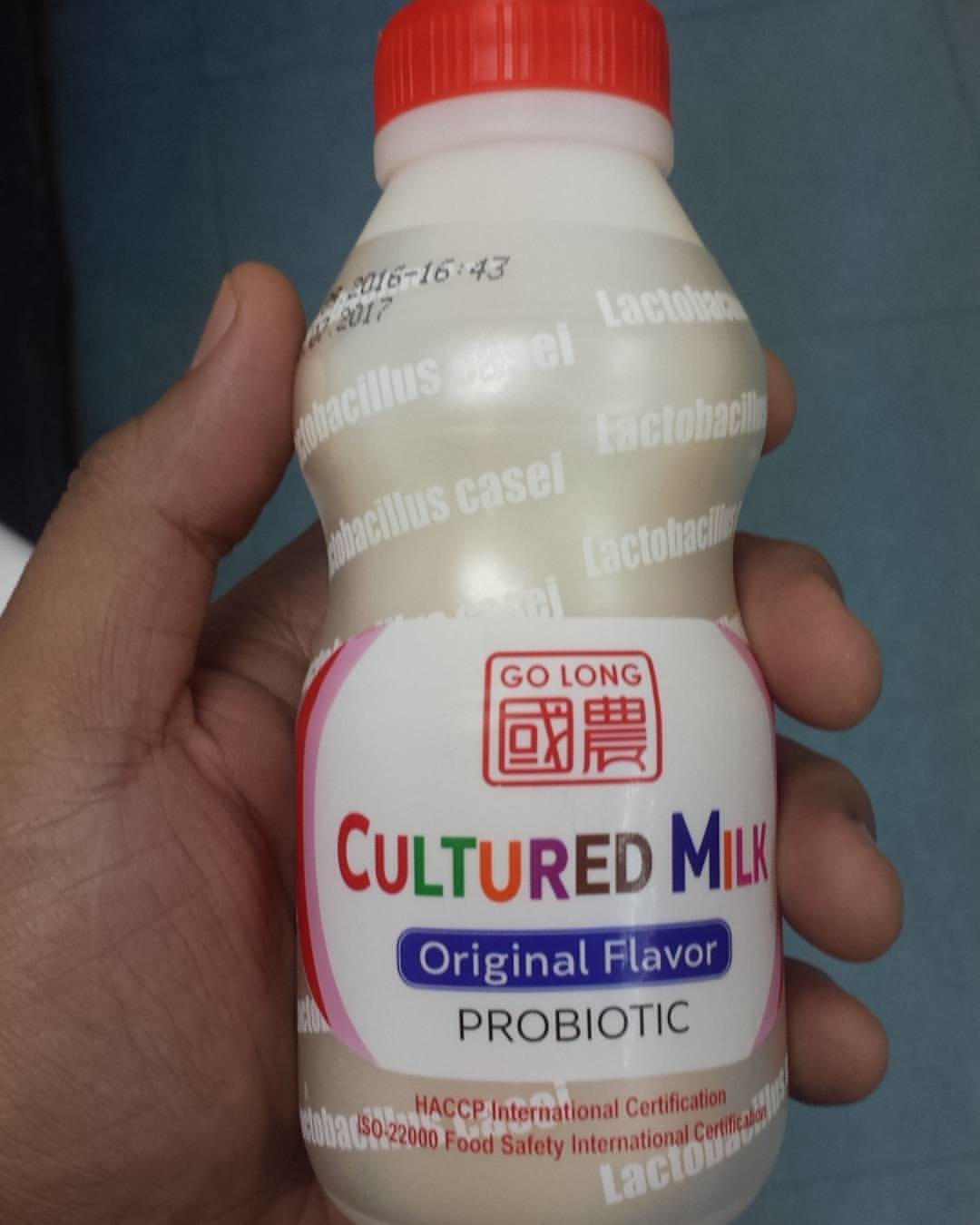In the photograph, a white male hand is prominently featured, holding a drink bottle in its left hand, with fingertips wrapped around it and the thumb resting on its side. The bottle's design is striking, with a predominantly white and silver color scheme and a red cap. The bottle itself appears small, just slightly larger than the hand holding it. The upper part of the bottle is white, transitioning to silver for the label that covers about two-thirds of its length. The label features a mix of detailed text and vibrant colors: it prominently displays the words "Lactobacillus Casei" and "Go Long" in a red box, alongside the phrase "cultured milk" with each letter in different colors—ranging from red, pink, green, orange, to purple and other hues.

Beneath the colorful text, there's a blue box with "original flavor" written in white, followed by "probiotic" in black. The bottle also mentions certifications such as "HACCP international certification" and "ISO-22000 food safety international certification." Notable numbers like "2017" and "2016 1643" appear on the left. The entire scene is set against a neutral blue or gray background, making the intricate details and colors on the bottle stand out vividly.